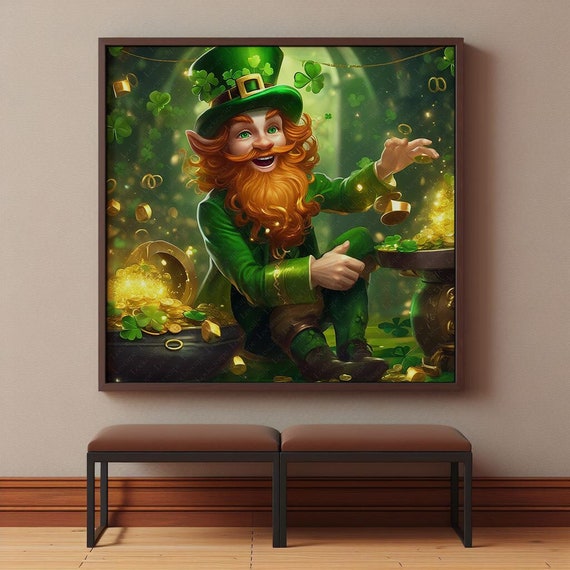The image depicts an indoor scene, possibly a hallway or waiting room, characterized by light brown, beige-colored walls and a light wood tile floor. Centrally mounted on the wall is a large, square piece of cartoony artwork in a dark wood frame. The artwork portrays a leprechaun with human-like features, including a long reddish-brown beard, mustache, and bushy eyebrows. The leprechaun, wearing a green outfit with gold trim and a green hat adorned with a gold buckle, is seated with his knees up, smiling with his mouth open. He holds an unidentified gold object in his hand as various items, like shamrocks and pieces of gold, float around him. Below this framed artwork are two side-by-side benches with black legs and brown or dark red seat cushions. The scene is further framed by a tall brown baseboard skirting the bottom of the wall.